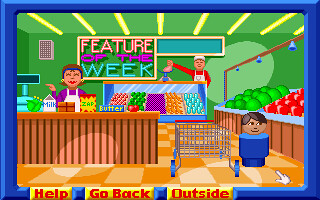The image, a screenshot from a video game, features a vibrant and cartoony depiction of a supermarket scene. The entire screen is framed by a royal blue outline, with three yellow rectangular options at the bottom labeled "Help," "Go Back," and "Outside." The background walls and ceiling are green, and the ceiling is fitted with yellow lighting fixtures. 

In the foreground, a brown checkout counter with black stripes houses a green cash register. Behind the counter stands a female cashier dressed in a purple shirt and a white apron. On the counter are various products: an apple, a stick of butter, a red box labeled "Zap," a carton of milk, and possibly a head of lettuce. A shopping cart is positioned nearby with a character that has a simplistic, cylindrical body resembling a Lego figure, featuring a light brown circle face and dark hair.

To the right, there are displays of watermelons and red fruits, perhaps apples, arranged in brown wooden stands. In the background, a man dressed in a red shirt, red apron, white hat, and white apron stands next to a deli counter, holding up a piece of meat with his outstretched arm. Behind him is a prominently displayed banner that reads "Feature of the Week" in bright, multicolored text with a peach and pink font, bordered by a yellow-tan color. The scene is lively and bustling, accurately capturing a typical day at a busy supermarket in a charming, animated style.